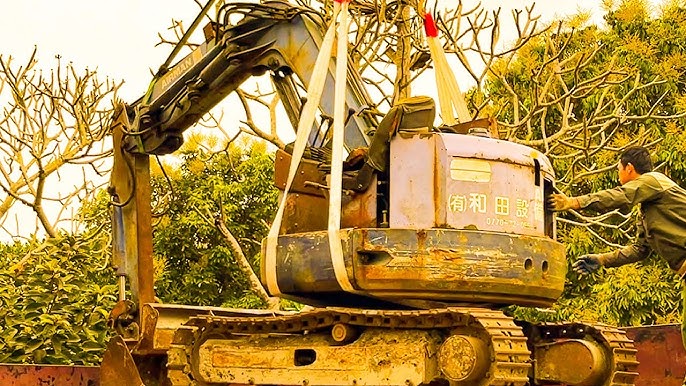In the picture, a smaller-sized, weathered bucket loader with rusty yellow paint and an extended crane arm is being hoisted by tow straps from a red trailer. This piece of construction equipment, equipped with small tracks on either side and a seat for the operator in the swivel area, features Asian characters—likely Chinese or Japanese—on its back. A man, whose hands appear dirty or stained with oil, is positioned at the rear of the machine, ensuring its safe handling as it is lifted. The background reveals a lush, green forest indicative of summertime, contrasting with a few sparse trees that are barren of leaves.